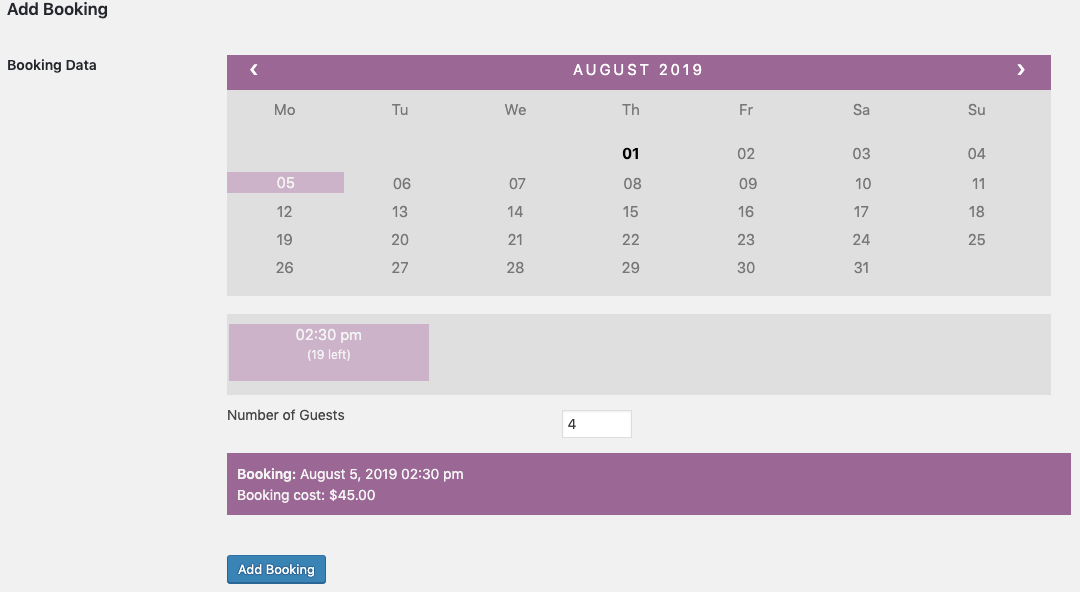This is a webpage for booking accommodations or events. The interface features a clean design with a primary focus on usability. 

At the top, there is a prominent gray box with black text that introduces the booking section. Below, there is a lavender header that stands out with a slightly darker gray background, drawing attention to the key interactive elements. The title "Ad Booking" is positioned at the top-left corner, followed by "Booking Data" underneath. 

This section features navigational arrows on either side, allowing users to browse through different dates. The current displayed date is set to August 5th, 2019.

Underneath the date navigator, there are columns for each day of the week: Monday, Tuesday, Wednesday, Thursday, Friday, Saturday, and Sunday. The calendar grid below these headers displays the days of the month, ranging from 1 to 31.

Focusing on August 5th, 2019, there is a highlighted bar in lavender that indicates the time frame of 12:00 PM to 12:30 PM. The exact time slot isn't completely clear but provides a visual cue for the selected booking time. 

Below the time slot, the interface includes a section to specify the number of guests, defaulting to 4 guests. Following this is another lavender box that reiterates the booking details: "Bookings: August 5, 2019, 12:00 PM to 12:30 PM."

Further down, the cost of the booking is clearly stated as $45. A blue clickable tab labeled "Add Booking" allows users to finalize their reservation for the specified date and time. 

Overall, the page is structured to offer a straightforward and user-friendly booking experience for the specified date of August 5th, 2019.